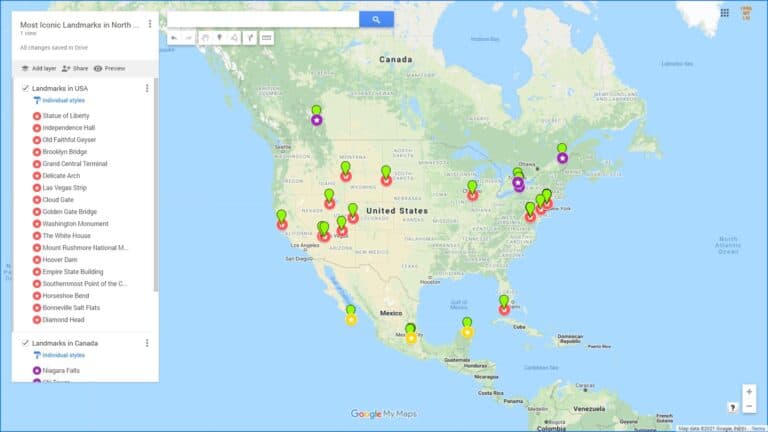The image depicts a detailed map highlighting numerous iconic landmarks across North America. Key landmarks in the United States are prominently marked with colored pins, including:

- The Statue of Liberty in New York
- Independence Hall in Philadelphia
- The Brooklyn Bridge in New York
- Grand Central Terminal in New York
- Mount Rushmore National Memorial in South Dakota
- The Empire State Building in New York

Additionally, geographic locations such as the notable areas of the Southern Bronx and Portland are also indicated. In Canada, specific landmarks and general locations are marked, with the Bay Area notably marked and lush grasses depicted. The map features a green pin and a purple pin among various locations.

The map also includes markers in Mexico, showing three distinct pins for important sites. The pins are numbered consecutively, indicating 11 significant locations in the United States. In contrast, three major sites are marked in Mexico. Furthermore, the map displays textual elements such as "North Atlantic Ocean" and various annotations in the bottom right corner, providing additional geographical context.